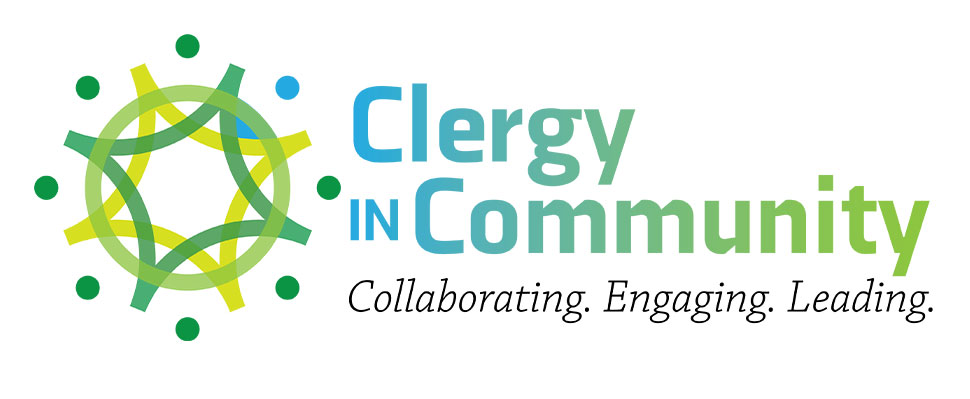The image features the logo of an organization named "Clergy and Community" on a white background. The logo is a circular design incorporating two overlapping curved squares in shades of green, with an inner curved square in mustard yellow. To the left of these shapes is a blue dot, encircled by numerous green dots that surround the entire logo. Below the organization's name, the words "Collaborating, Engaging, Leading" are displayed, each followed by a period. The overall layout appears clean and upright, emphasizing the theme of community collaboration and leadership through a harmonious mix of green, yellow, and blue elements.